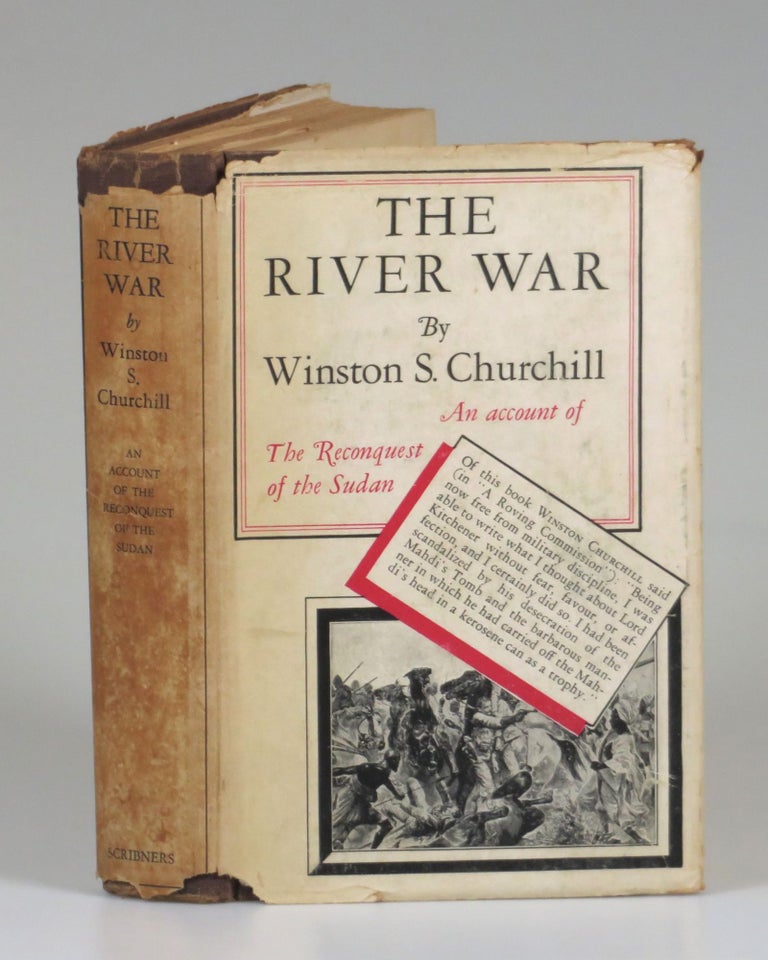This photograph showcases an old, hardcovered book titled "The River War" by Winston S. Churchill, recounting the reconquest of the Sudan. The cover and spine of the book are visible, reflecting its age with worn, torn edges and discolored, cracked fabric binding. The title is prominently displayed in a mix of black and red fonts, enclosed in a black square with a red border. Below this title square, there's a black-and-white, framed, wartime image of men, including one holding a gun. Between these visual elements, there's a skewed black rectangle layered on a red background featuring a quote from Churchill, stating: "Being now free from military discipline, I was able to write what I thought about Lord Kitchener without fear, favor, or affection, and I certainly did so. I had been scandalized by his desecration of the Mahdi's tomb and the barbarous manner in which he had carried off the Mahdi's head in a kerosene can as a trophy." This detailed excerpt emphasizes Churchill's critical view of Lord Kitchener. The book's pages appear old and yellowed, adding to its historical aura.